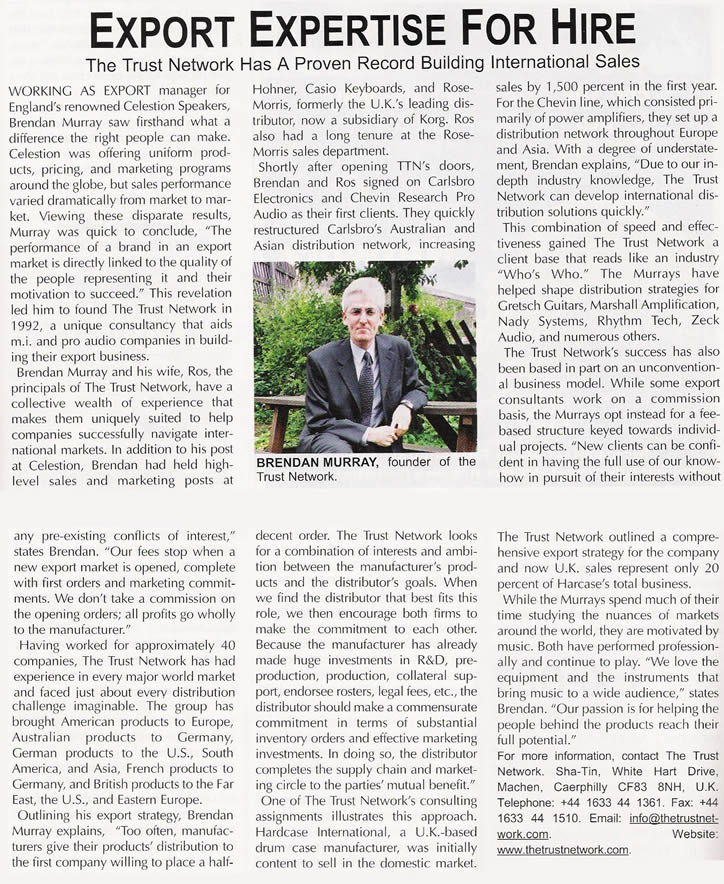This image appears to be a layout from a newspaper website. The page features a light grayish background with a classic newspaper design aesthetic. The headline at the top of the page is in large, bold, black, all-capital letters, with the first letter of each word slightly larger than the others, reading: "Expert and Expertise for Hire." Below the headline, in a slightly smaller but still emphatic font, a subheading states: "The Trust Network Has a Proven Record Building International Sales," with every first letter capitalized.

The content is organized into three columns that extend halfway down the page, followed by a small space, and then another set of three columns. Located about halfway down the second column of the top section, there is a photograph of a man sitting outside on a brown bench, with a large bush and some lights in the background. The man, dressed in a suit, has white hair and is posed with his left elbow resting on the bench and his other arm across his lap. Beneath the photograph, a bold, all-capitalized caption reads: "BRENDAN MURRAY," followed by regular text stating "founder of the Trust Network."

The articles and information continue to elaborate on the topic, filling the columns with detailed content. The layout includes a section at the bottom with the final paragraph inviting readers for more information. It provides contact details for the Trust Network, including an address, telephone number, fax number, email, and a clickable website link.